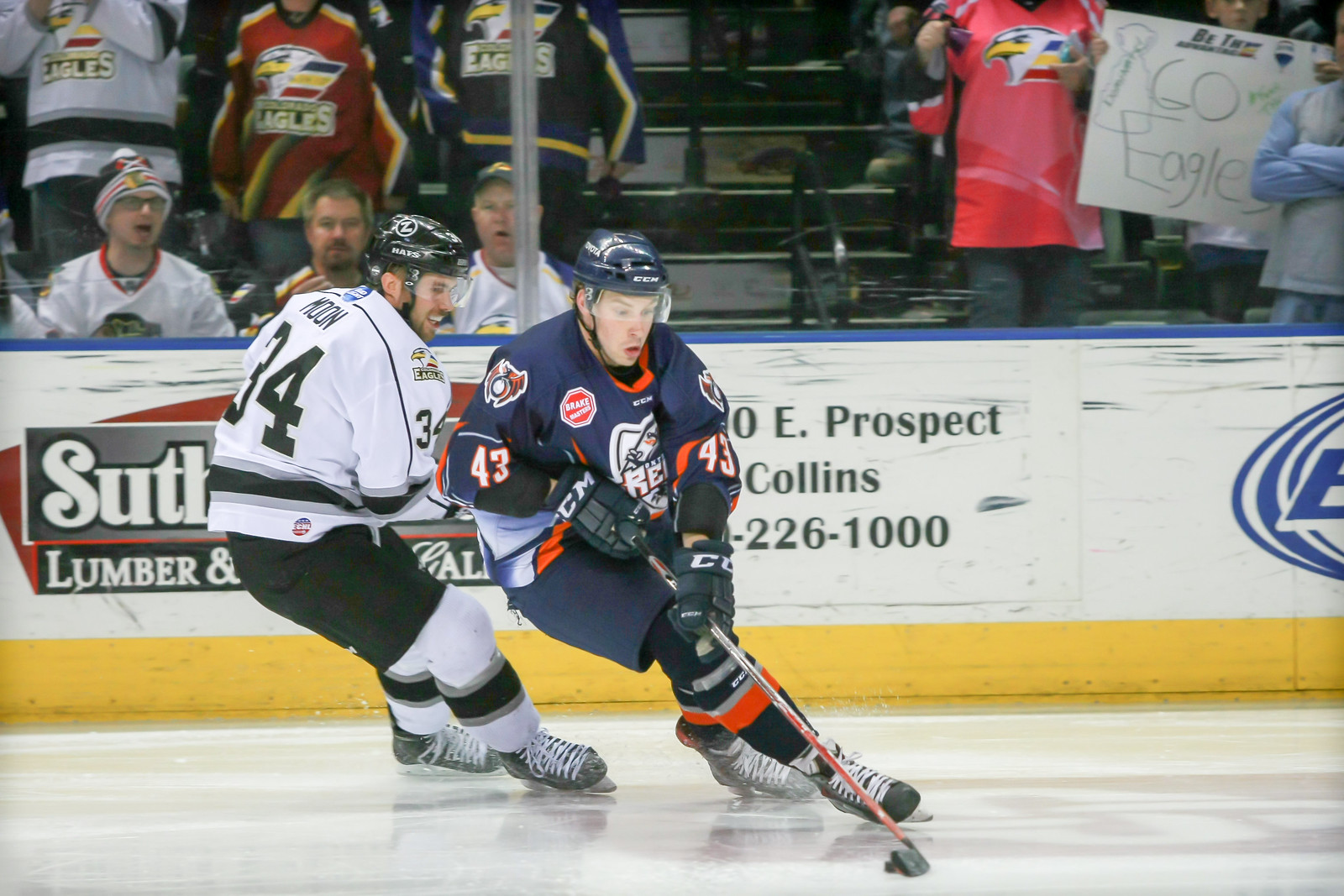In this dynamic ice hockey scene, two players are at the center of the action. The player in the foreground, dressed in a dark blue uniform, is skating from right to left with the puck expertly controlled by his hockey stick. He is a white male, mid-20s, with a helmet securely in place. His blue jersey displays the number 43 in white lettering on the sleeve, and although a large emblem on his chest is partially obscured by his arms, it’s clear he belongs to the home team.

Chasing him is an opposing player in a white jersey with the number 34 and the name "Moon" clearly visible. This player is also a white male, around mid-20s, with a black helmet, black pants, and white shoes atop gray skates. The word "Eagles" is prominently displayed on his right shoulder. Both players are intensely focused, leaning slightly left, with the player in white trying to catch up.

Surrounding the rink, the atmosphere buzzes with excitement. Fans are visible through the protective glass barrier, which sits above the boards marked with a yellow stripe at the bottom. The boards also feature ads, including a partially obscured Sutherland Lumber advertisement and fragments of another one showing "East Prospect Collins" and a phone number ending in “226 1000”.

In the stands, packed with viewers, several fans sport Eagles jerseys, clearly supporting the visiting team. A sign held up reads "Go Eagles," and near it, a woman stands out in a red shirt with an eagle emblem. Amidst the crowd, three men, likely in their mid-30s to 40s, are sitting, watching the game with intense interest. The fans are warmly dressed, indicative of the chilly rink environment, with a mix of hats and bare heads.

The smooth ice at the bottom of the photo reflects the glimmers of the action above, capturing the fast pace and intensity of this professional hockey match.